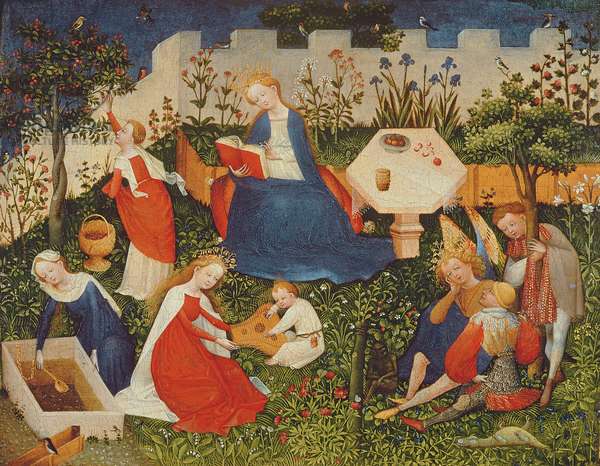The artwork depicted in the image is a detailed medieval painting capturing a bustling courtyard scene within a castle's stone wall that boasts notches and is adorned with colorful birds. The courtyard, rich in lush greenery, features an array of trees and an abundance of red and blue flowers amidst detailed grass, leaves, and branches. 

In the scene, a group of mostly women and children, along with a few men, engage in various activities. A woman in a blue dress sits reading a book, while another woman is seen picking something from a tree, likely fruit. Another female figure is busy digging in a rectangular box, possibly for planting. Nearby, a woman is either playing a musical instrument with a child or entertaining a baby with some device. 

Elsewhere, a man converses with two women or perhaps a man and a woman, and one person is lying on the ground while another sits and observes. One man looks up at the sky, and another gazes downward towards the grass. Additionally, there is an assortment of items on a table, including food, a cup, and a glass, indicating a springtime or leisure setting where people are occupied yet relaxed, immersed in the vibrancy of the garden.